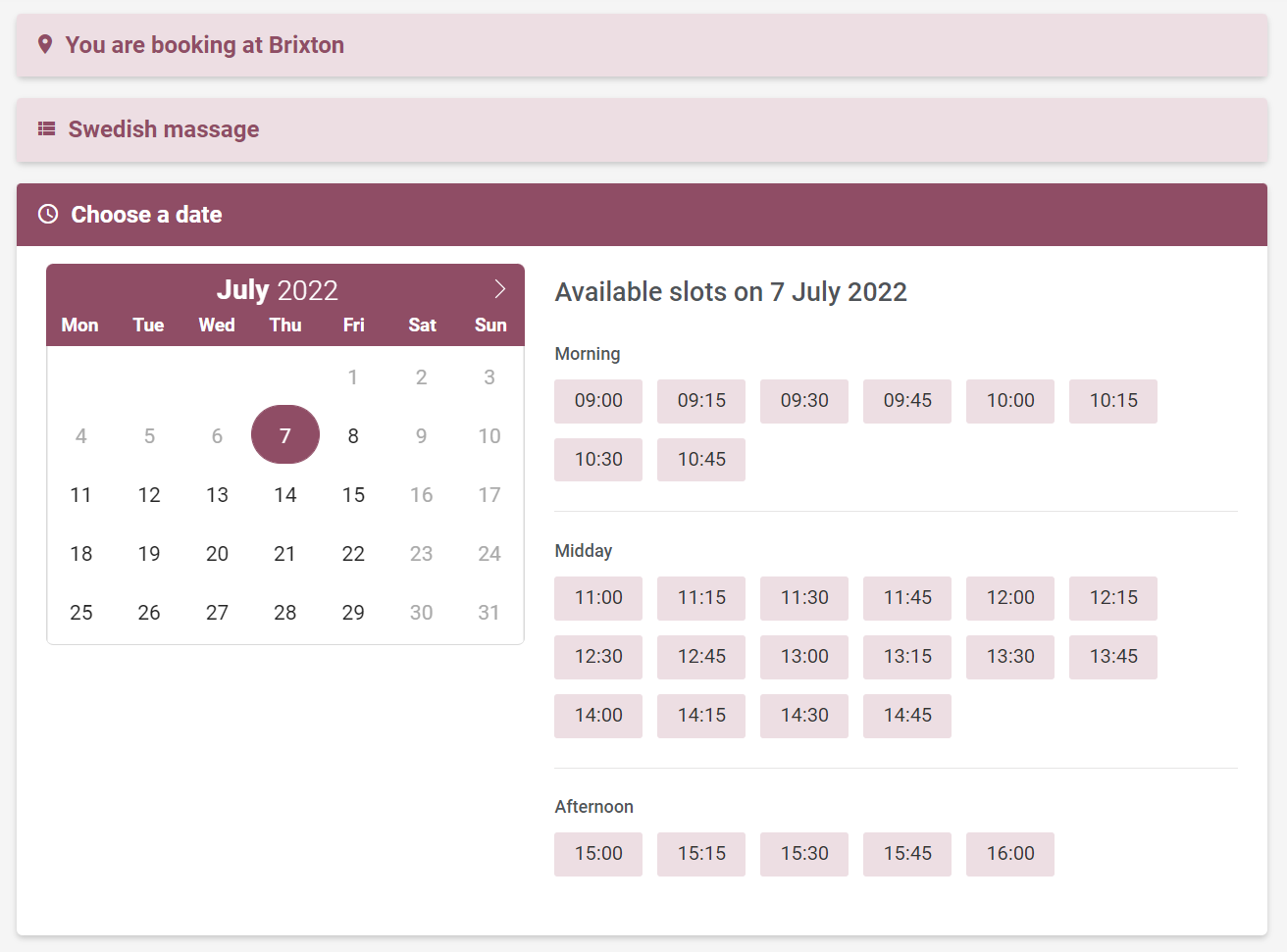Screenshot of a website for booking a service at Brixton. The user has navigated to the Swedish Massage booking section. On the left side, a calendar is displayed showing July 2022, with Thursday, July 7th selected. On the right side, the available time slots for July 7, 2022, are presented, divided into three categories: morning, midday, and afternoon. The morning slots range from 9:00 AM to 10:45 AM, midday slots from 11:00 AM to 2:45 PM, and the afternoon slots from 3:00 PM to 4:00 PM.